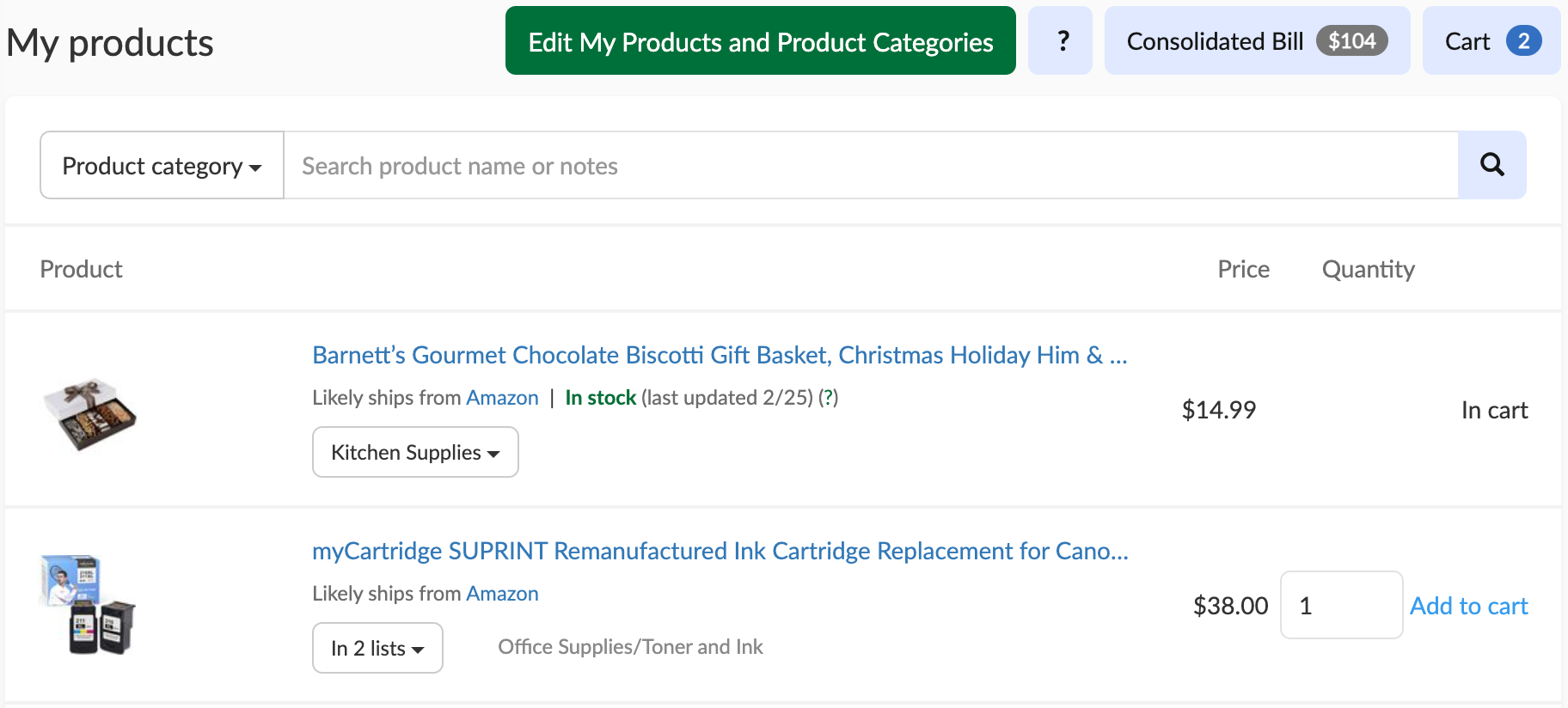Screenshot of My Products Interface:

The image showcases the "My Products" interface, featuring a sleek, white-box design. In the upper left-hand corner, the title "My Products" is prominently displayed in bold, black text. Directly to the right, there is a green button with a white font, labeled "Edit My Products" and "Product Categories," suggesting it offers clickable options. Adjacent to this, a light blue button with a question mark icon indicates available help or support resources.

Further along the top bar, another blue button labeled "Consolidated Bill, $104" appears clickable, likely for viewing billing information. Next, an icon representing a shopping cart shows the number "2," signifying that there are two items currently in the cart.

The main section of the screenshot contains a search functionality, starting with a dropdown menu on the left labeled "Product Category," which users can presumably adjust to other options like "Product Name." A search box allows for input of "Search Product Name or Notes." Beside this, another question mark icon implies assistance is available.

Displayed beneath the search area are two product listings:
1. "Barnett's Gourmet Chocolate Biscotti Gift Basket, Christmas Holiday Hymn," which specifies it ships from Amazon, is noted to be in stock, and is priced at $14.99.
2. "My Cartridge Superhint Remanufactured Ink Cartridges Replacement," also indicating it ships from Amazon, priced at $38. An option to the right side of this listing suggests adding the item to the cart. 

All visual cues and functionalities are clearly designed to guide the user through managing and purchasing their products seamlessly.